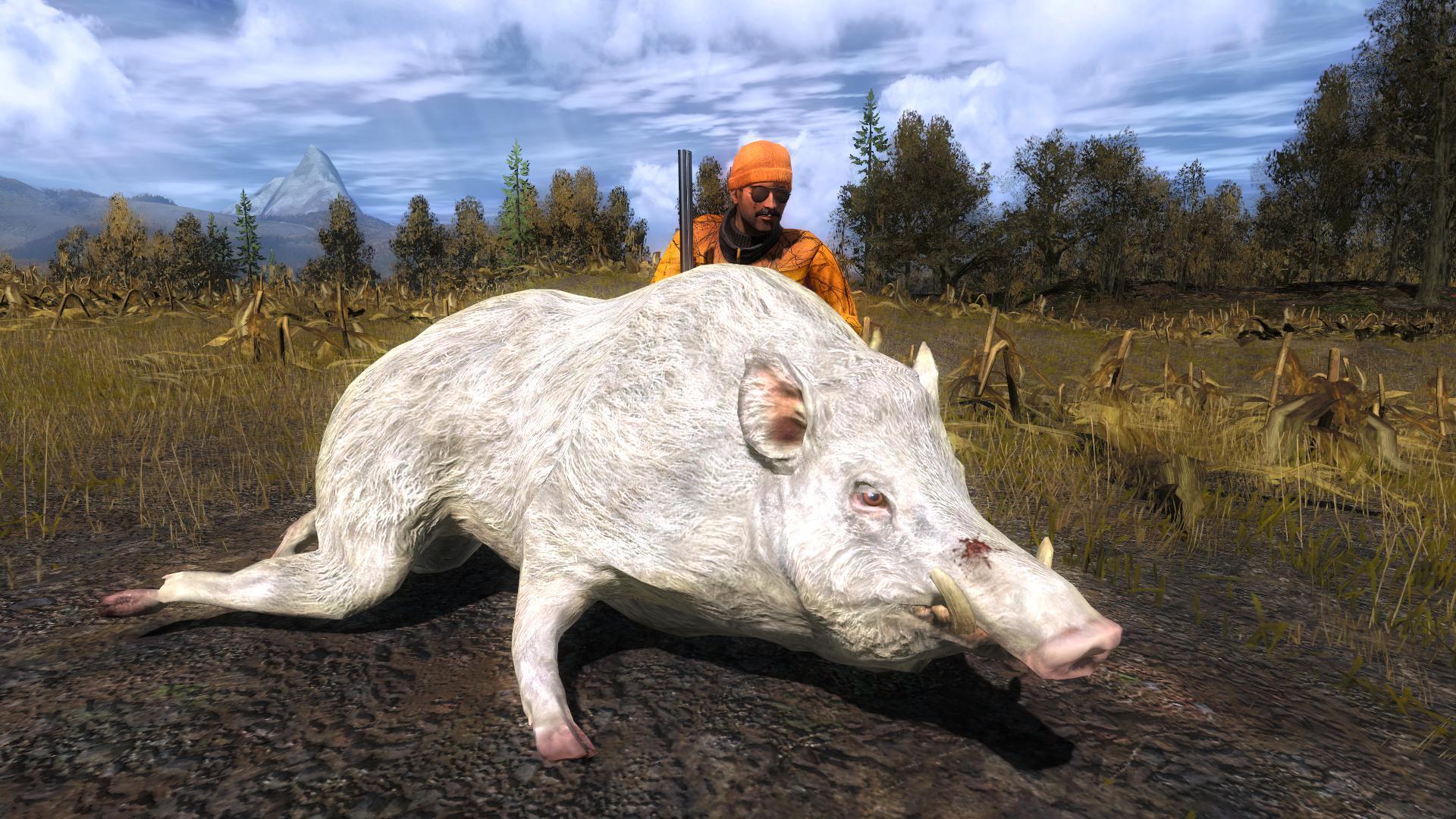This detailed photograph captures a hunter kneeling behind a large, white wild boar he has presumably shot. The hunter, wearing a bright orange hat, orange and black hunting jacket, and sunglasses, holds a double-barrel rifle resting on his shoulder. The wild boar, which takes up most of the frame, is distinctly white with pink ears, a pink nose, and pink hooves, as well as small tusks protruding from its mouth and hints of pink around its eyes. There's a notable blood splatter on the ridge of its nose. The boar is positioned centrally on the muddy ground, its forelegs slightly extended outward, and is facing right at a three-quarter view angle.

The scene is set outdoors in a large field with a dirt or muddy area in the foreground. Behind the boar, a row of tall green trees stretches across the background, with a mountain peak visible to the left. Above, the sky is bright blue with a mix of white puffy clouds. The overall atmosphere of the photograph is natural and serene, with no text associated with the image. The field extends towards the tree line, giving way to tall grass or corn stalks, creating a layered visual from the muddy foreground to the towering backdrop.